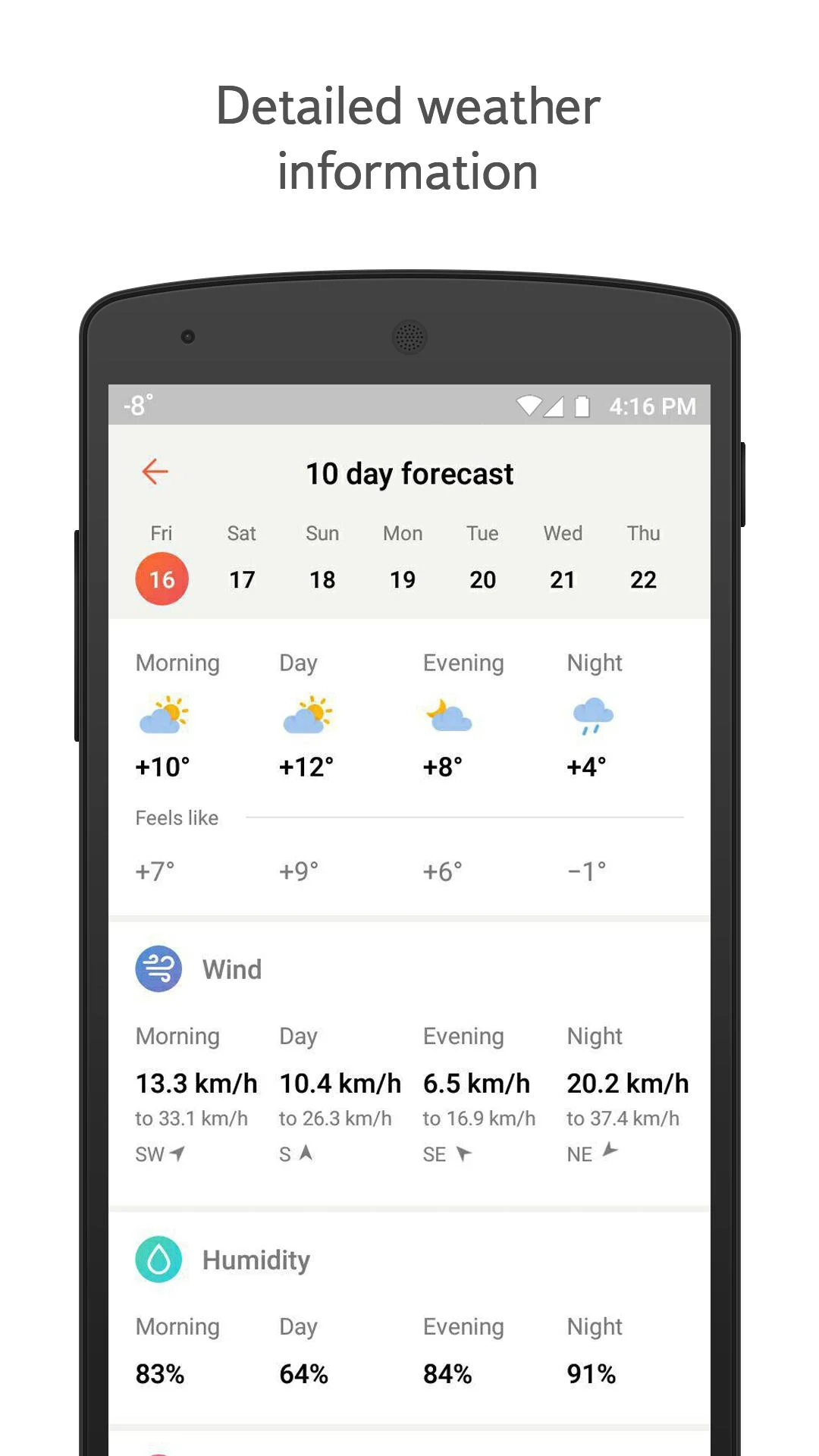The image shows a detailed 10-day weather forecast displayed on a tall smartphone, characterized by its predominantly light theme with shades of gray and white, and a slim black border. The forecast spans from Friday to the following Thursday, covering dates from the 16th to the 22nd. Each day has segmented predictions for morning, day, evening, and night, depicting varying weather conditions such as clouds and sun.

Friday predicts cloudy weather with temperatures ranging from a high of 10 degrees to a low of 4 degrees, and it feels like temperatures between 7 degrees and -1 degrees. Wind speeds fluctuate throughout the day, with morning winds from the southwest at 13.3 to 33.1 kilometers per hour, southward winds during the day at 10.4 to 26.3 kilometers per hour, southeast winds in the evening reaching 6.1 to 60.9 kilometers per hour, and night winds averaging 20.2 to 37.4 kilometers per hour from an unspecified direction.

Humidity levels change as the day progresses, starting at 3 percent in the morning, rising to 64 percent during the day, 84 percent in the evening, and peaking at 91 percent at night. The rest of the days appear to follow similar detailed patterns of weather prediction, providing comprehensive information for each part of the day.

Overall, the forecast is clear and user-friendly, with distinct sections for different weather elements. The smartphone's light theme enhances readability, making it easy to glance at all the essential weather details for careful planning.